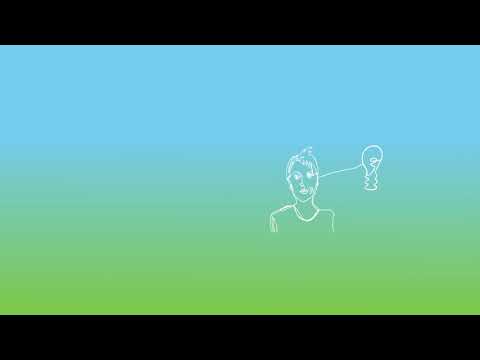The image is a smaller, horizontally-aligned rectangle with thick black borders at the top and bottom. The central background transitions from a light blue at the top to green at the bottom in a smooth gradient. Near the center-right, there is a white, outlined drawing of a person's head and shoulder, wearing a shirt with a round collar. This figure, which appears to be male with short hair, has detailed features including white-colored eyes and a mouth. Extending diagonally from the person's head to the right is a white line that connects to an outline of a light bulb. The predominantly used colors in this image are black, white, light blue, and green, and it appears to be a digital drawing with no accompanying text.